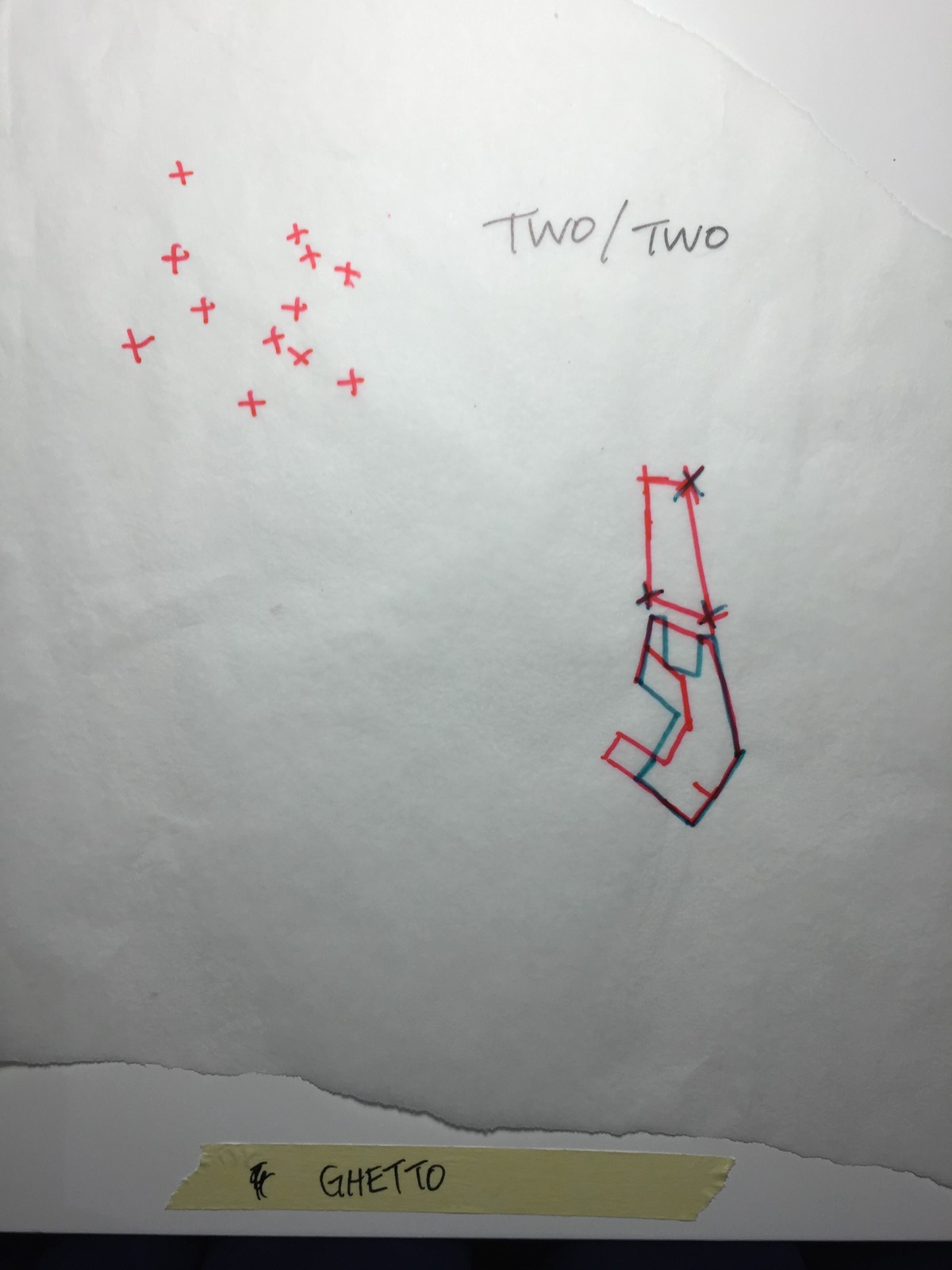This detailed caption describes an artwork:

A vivid, mixed-media artwork mounted on a white piece of paper, hanging on a wall. The top of the paper features the text "2/2" prominently displayed in all caps, written in black ink. Adjacent to this text are several red X's, seemingly sketched with a bold magic marker. Below this, on the lower right portion of the page, there is a layered geometric composition. The base layer is a red trapezoid-like shape. Overlaying this red foundation, there is a blue shape that roughly mirrors the red one but extends into a C or U configuration with a connecting line. Sprinkled atop the red shape are a few blue X's, adding further texture. Affixed to the bottom of the paper is a piece of yellow tape with the word "Ghetto" inscribed in black ink, serving as a striking caption and further embedding the image into the surrounding context. The entire assembly is fastened to the wall, creating an engaging visual statement.